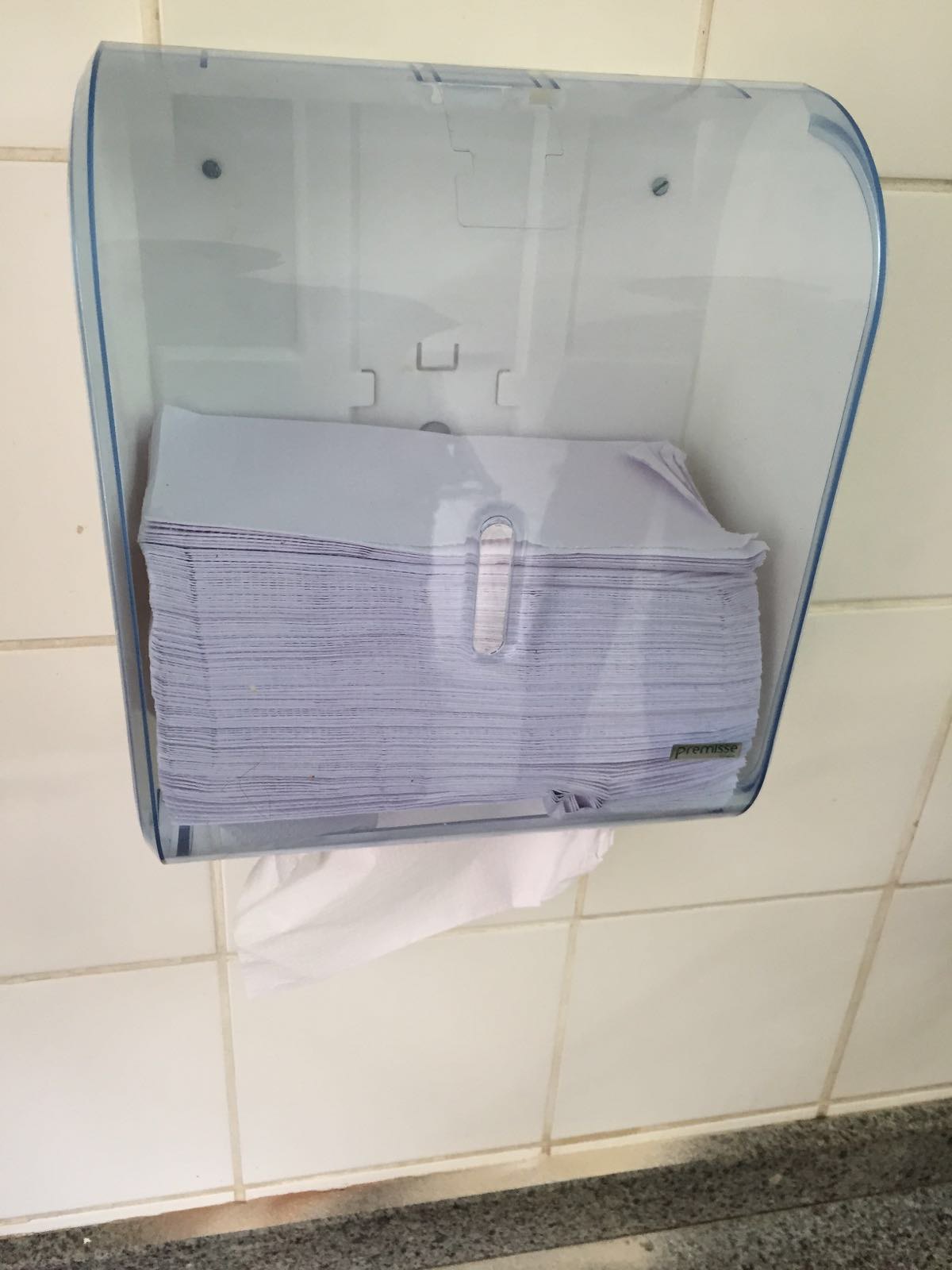The image features a blue-tinted, transparent plastic napkin holder attached to a white tile wall with visible grout lines. The napkin holder, which has a curved top and an oval hole in the center, is halfway filled with white, tri-fold napkins reminiscent of those found in public restrooms. Below the napkin holder, a black and gray speckled countertop with a metallic border is partially visible. Reflections on the plastic surface of the napkin holder obscure some details but add dimension to the image. The overall scene suggests a utilitarian setting, possibly a kitchen or a public restroom, emphasizing the practicality and visibility of the napkin holder filled with functional paper towels.